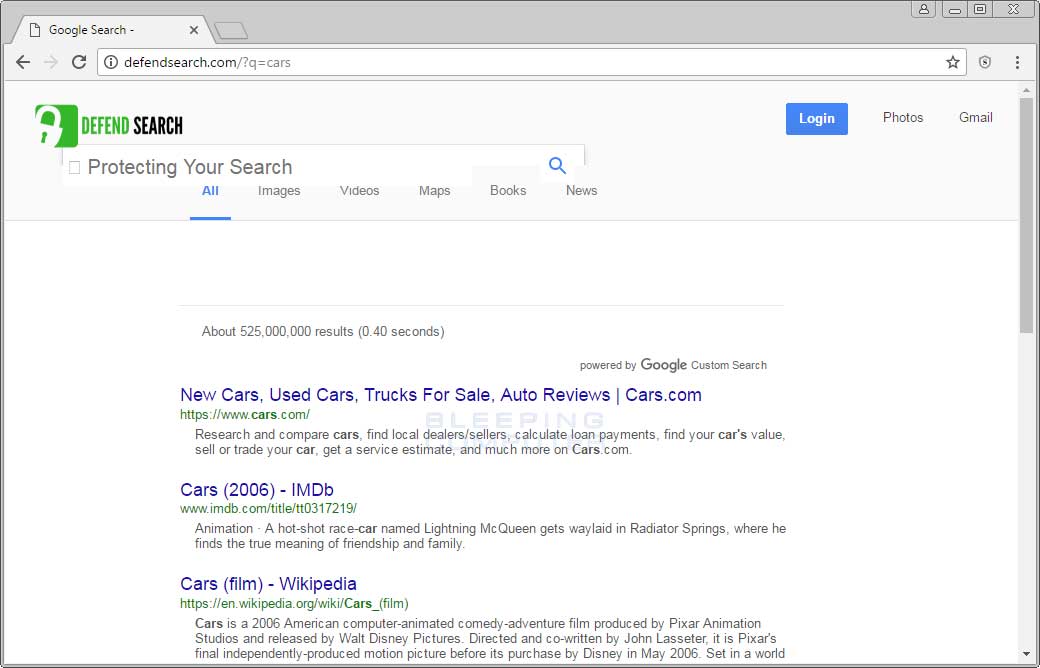This image is a screenshot of a web browser window. The top bar is gray, displaying a person icon, a minimize button, a maximize button, and a close button (X), all in white with gray outlines, positioned on the top right. 

There is a single tab open titled "Google Search," represented by a small document icon with a folded top corner. Below the tab, the navigation bar is displayed, containing a series of control elements: a left-pointing gray arrow, a lighter gray right-pointing arrow, a darker gray refresh button, and a URL field. The URL shown is "defense-search.com/?Q=cars", with an 'i' inside a circle symbol preceding it. To the right of the URL box, there are three icons: a gray outlined star, a shield icon, and a vertical stack of three dots.

The website being viewed is labeled "Defend Search," indicated by a green icon with a lock symbol. The text "Defend" is in green, while "Search" is in black. Adjacent to this, there is a blue "Login" button and options for "Photos" and "Gmail" displayed in gray text within a light gray box. Below this header, there is a search bar displaying a blue magnifying glass icon and the phrase "Protecting your search."

The search results are laid out below the search bar, featuring links in blue text, their URLs in green, and descriptions in gray.